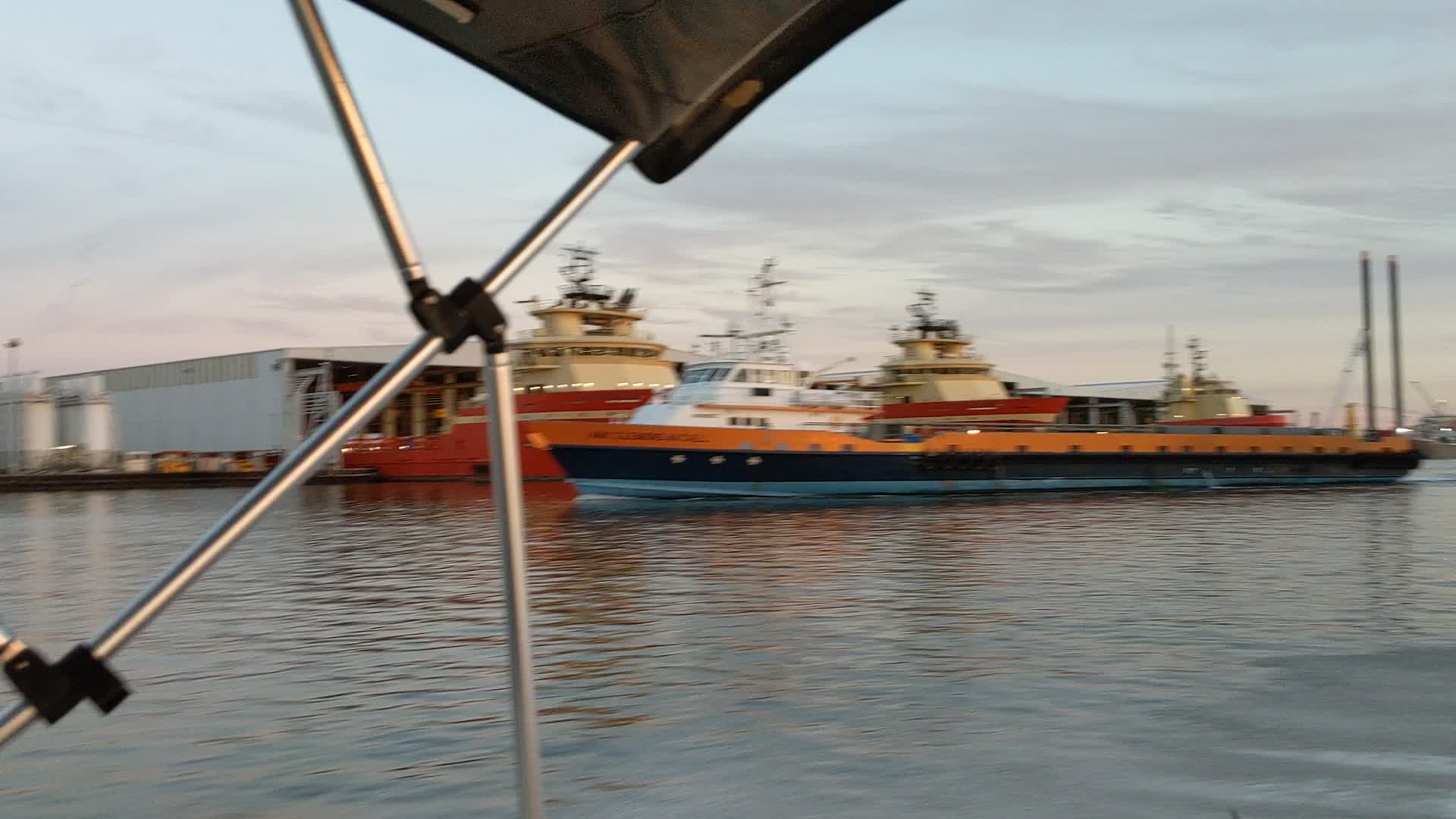The photograph captures a bustling port scene at dawn or dusk, marked by a pale blue sky with wispy clouds tinged with pink near the horizon. In the foreground, two large ships are prominently featured, floating on a greyish-blue expanse of water that reflects their vibrant colors. The primary vessel is an eye-catching combination of orange, dark blue, and light blue stripes with a white top. Just behind it, a large red and white ship looms, partially visible but no less imposing. Both ships are anchored near a dock adjacent to a large grey warehouse or structure. Adding to the scene's complexity, parts of a smaller boat, likely from where the photo was taken, intrude into the frame. These include some intersecting metal poles with black plastic joints and a square canopy, giving a glimpse of the mechanical features of the photographer's vantage point.